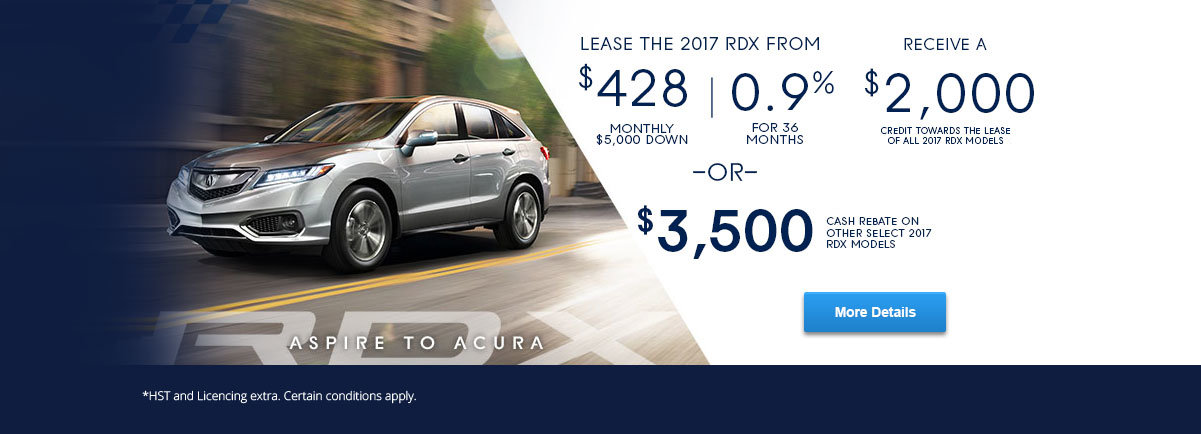This image is a detailed screenshot of an Acura website. Featured prominently is an image of an Acura sedan in a sleek light gray or silver color, identified as the Acura RDX. The text beneath the sedan reads "RDX," within which is the phrase "Aspire to Acura." Just below this, there’s a dark blue bar containing the text "HST and licensing extra conditions, certain conditions apply."

On the right side of the image, the screen is divided diagonally, separating the main image from a detailed section containing financing and leasing information for the 2017 RDX. The leasing information specifies that the 2017 RDX can be leased for $428 per month with a down payment of $5,000 for a duration of 36 months. Additionally, there is a special offer providing a $2,000 credit towards the lease of all 2017 RDX models. Alternatively, there is an option for a $3,500 cash rebate on other select 2017 RDX models, indicated in dark blue text.

At the bottom of this section, a light blue button with white text reads "More Details," inviting users to learn further specifics about the offers.